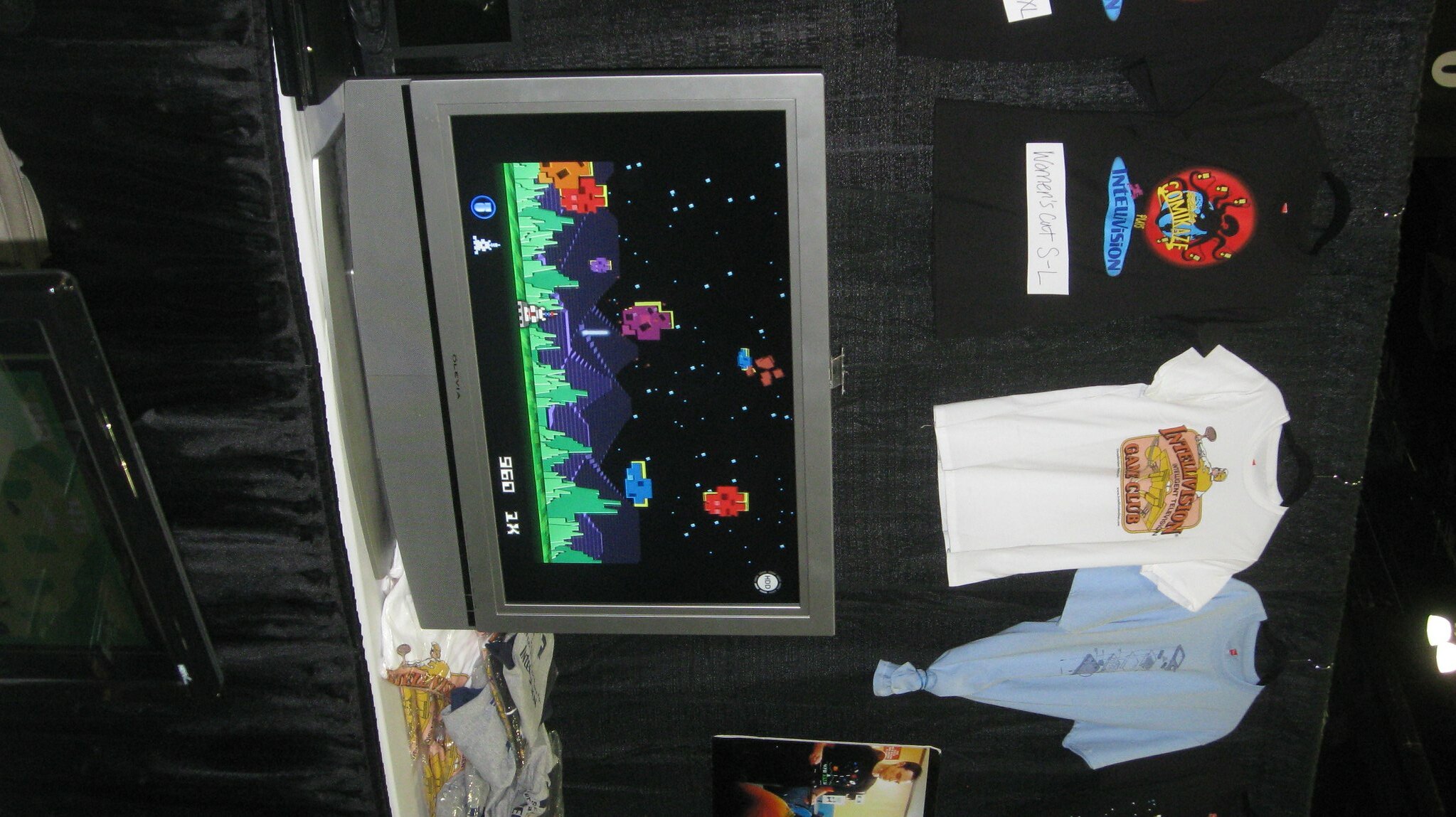This sideways-oriented photograph depicts a tech display booth or store setup. Central to the image is a silver Olevia television perched on a white table, showing a retro, pixelated space-themed video game. The game features a white spaceship at the bottom of the screen shooting at objects in a black sky, set against a green strip of land. Above the TV, a black curtain serves as a backdrop for several t-shirts suspended on metal hangers. Prominently displayed are three shirts: a black t-shirt with a red circular graphic and a small white paper detailing its size, a white t-shirt with a beige graphic including the words "Intellivision Game Club," and a blue t-shirt. A fourth shirt is partially visible in the upper right-hand corner. 

The setting suggests a vibrant mix of nostalgic gaming culture and merchandise, potentially part of a display booth at a tech conference or a specialized store.